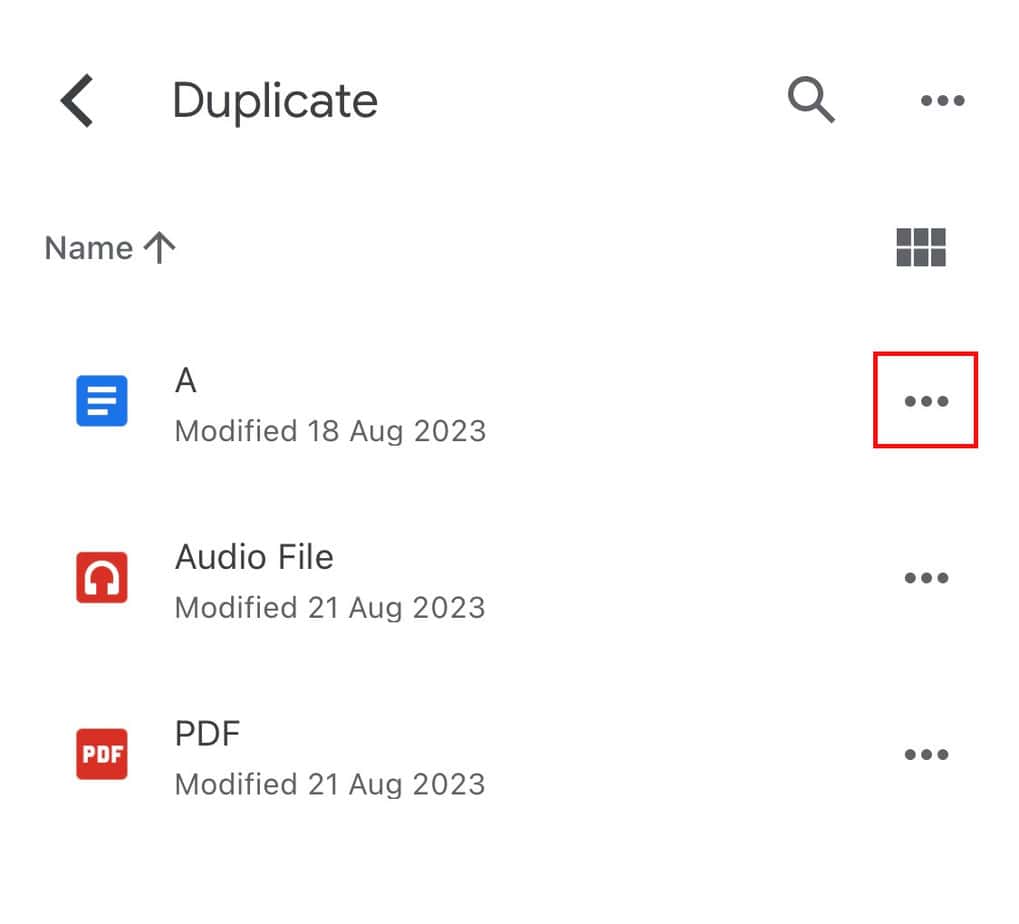The image features a clean, white background. At the top, a large, bold arrow points to the left with the word "duplicate" beside it. To the right of this arrow, there is an icon of a magnifying glass, followed by three horizontal gray dots.

In the next row, there is the word "name," accompanied by an upward-pointing arrow. To its right, there is a larger horizontal rectangle composed of six vertical rectangles, each separated by white space to form a grid pattern. Next to the grid, there is a blue square containing two flush-left white lines, with the bottom line being slightly shorter than the top one. Below this blue square is a capitalized letter "A." Underneath it, the text reads "modified 18 AUG 2023."

On the right side, three horizontal dots are selected within a red square.

Moving downward, we see a red square icon with headphones, labeled "audio file." Below this, it says "modified 21 AUG 2023," followed by another set of three horizontal gray dots on its right.

To the left, there's a red box labeled "PDF," with the text "PDF modified 21 AUG 2023" underneath it. To the right of this label, there are three horizontal gray dots.